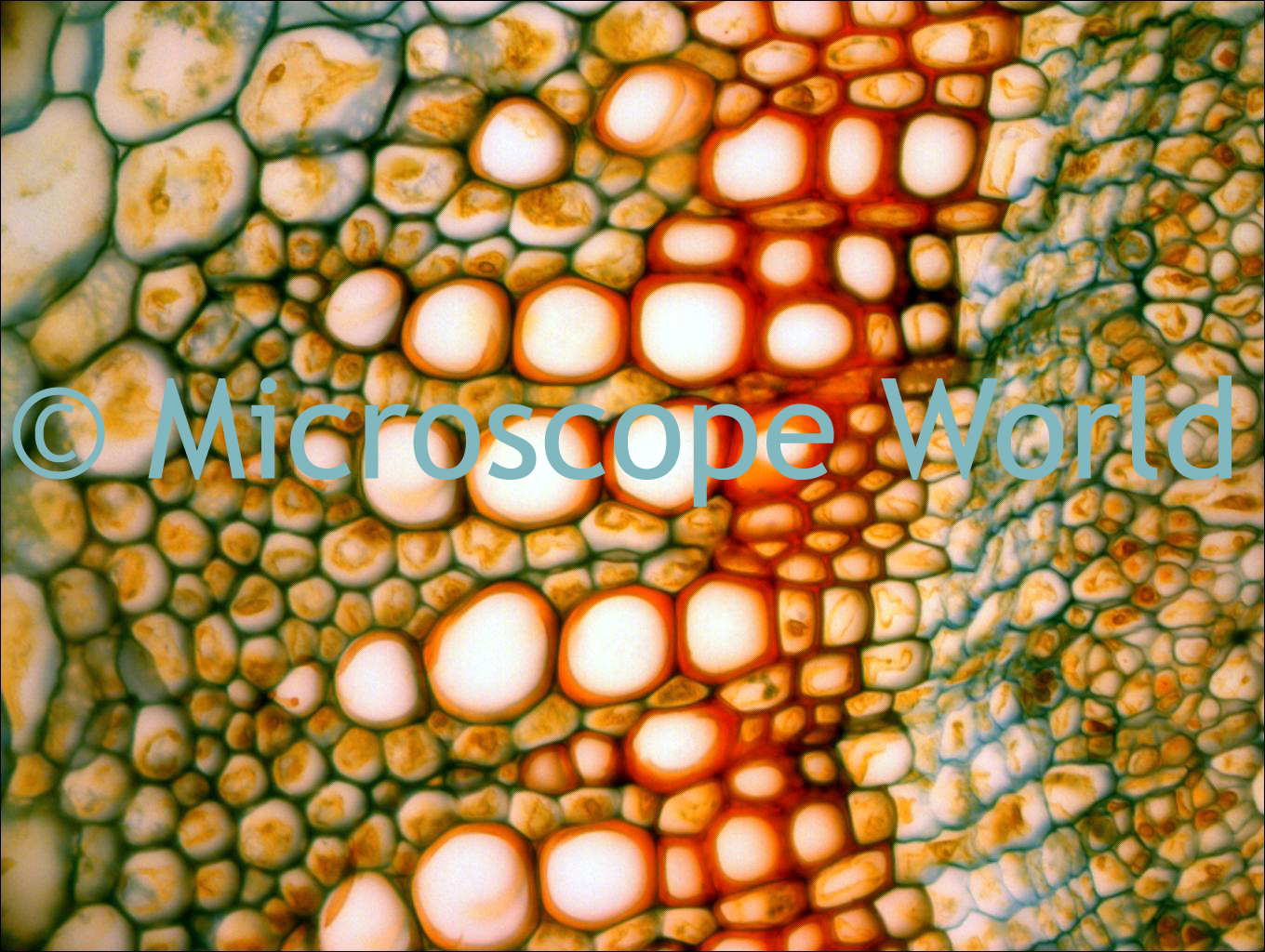This microscopic image, stamped with "Copyright Microscope World" in gray, showcases a vivid display of variously colored objects that resemble tiny pebbles or cells, arranged in distinct patterns and sizes. The scene primarily features objects in hues of red, yellow, green, and white, which transition in size from larger in the top left corner to smaller towards the edges. In the center, the colors predominantly merge into shades of red and white, surrounded by a mix of greens and yellows. Notably, the red and orange-rimmed white circles create an interconnected pattern, resembling cell linings or tightly packed elements akin to "corn on the cob." The detailed image also includes round objects with blue and brown elements, and quadrants of interlinking squares and circles, adding to the intricate design viewed under the microscope.